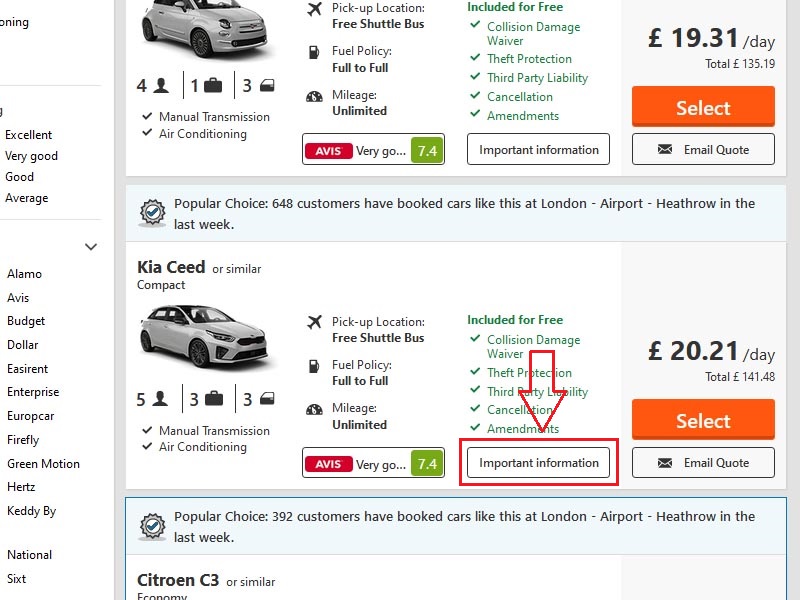The image is a partially cut-off screenshot from a car rental website, showcasing various car rental options. On the left, about two inches from the edge, it starts with a white background. The top left corner hosts incomplete text, "O-N-I-N-G," partially obscured. Below it is a list of ratings: "excellent," "very good," "good," and "average," all in black text, separated by a gray line. 

Beneath these, a list of car rental agencies such as Alamo, Agis, Budget, Dollar, and down to Keddy By Europcar, extends with a small gap that features "National" and "S-I-X-T." Continuing right into a light gray background, this section is divided into categories with headings at the top. Each category begins with a photo of a car, followed by details on its seating capacity, suitcase space, door count, annual transmissions, and air conditioning, indicated by checkmarks.

Additional information includes whether a shuttle bus service is available, fuel policy, and mileage limits. Below the car photo for Avis, a green box with white text gives its "very good" rating. Details of included amenities follow, alongside a clickable white tab with a black border labeled "important information." 

To the right, in a gray section, the price per day and total price are displayed with an orange "select" button in white text. Underneath, a white tab with a black border and an email icon invites users to "email quote." Below this entry, another car listing replicates the same formatting and information structure.